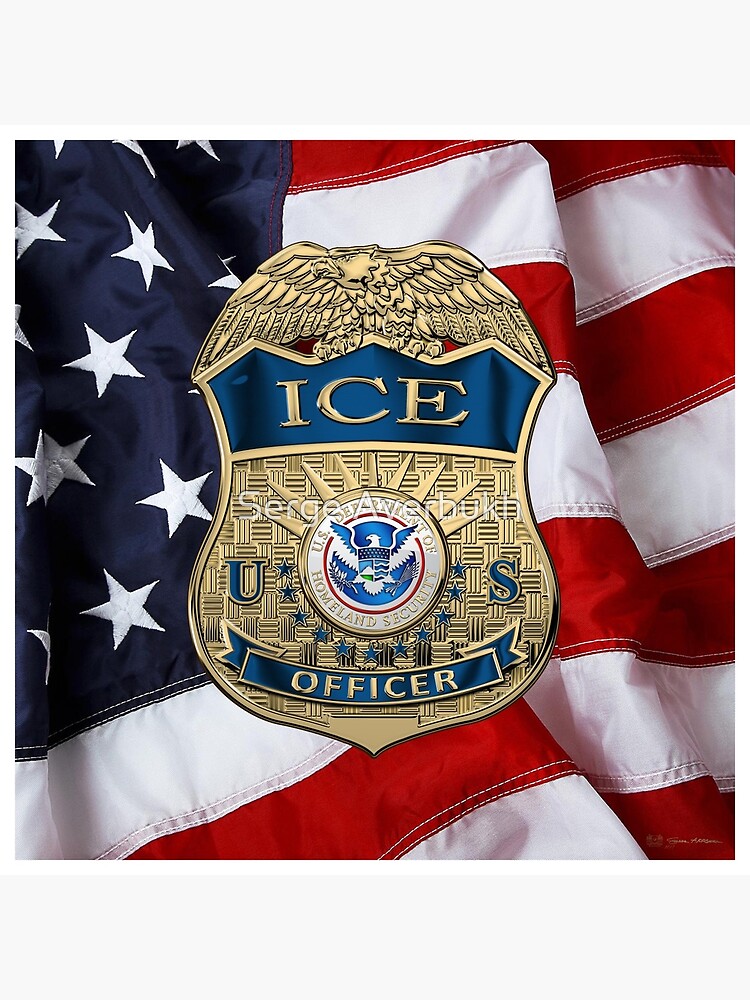The image features a detailed illustration of an ICE officer's badge set against a partially visible, realistic depiction of the American flag, with its dark blue field and white stars on the top left, and the red and white stripes on the right. The badge itself prominently displays a golden American eagle with outspread wings at the top. Below the eagle is a shield with a glossy dark blue upper section bearing the gold text "ICE," and a golden lower section featuring a detailed circular emblem. This emblem includes the seal of the U.S. Department of Homeland Security encircled by blue stars, flanked by a blue letter "U" on the left and an "S" on the right. A blue curved banner at the bottom of the badge bears the gold text "Officer." The badge also has a subtle white watermark reading "Serge Averbeck." The image combines photographic realism with illustrative elements, providing a clear and detailed portrayal of the badge and its symbolic background.